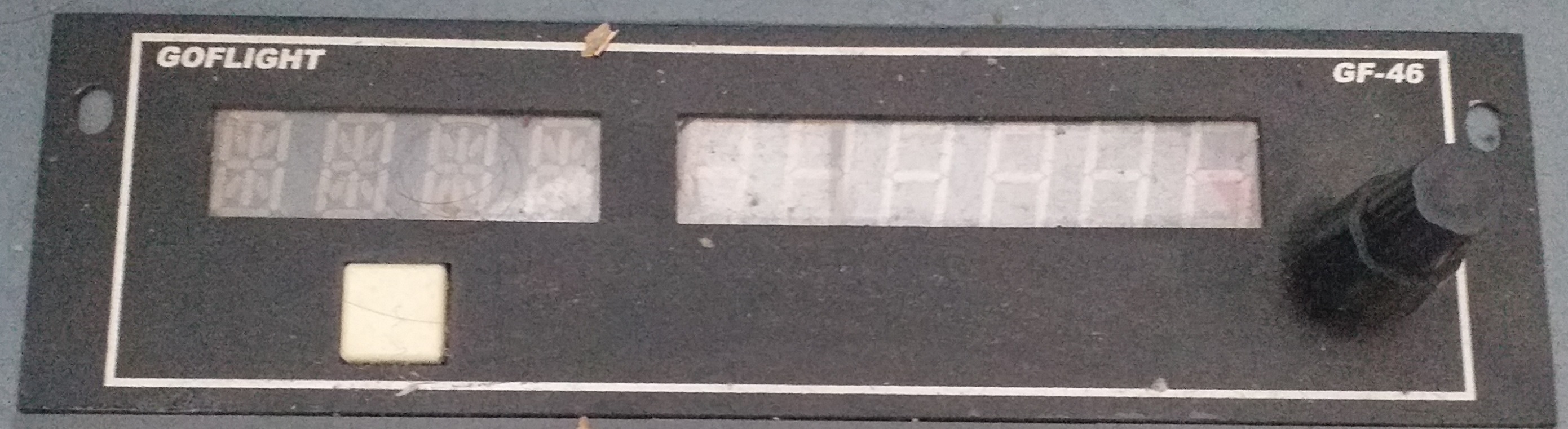In the image, we observe a sleek, flat black device made of metal featuring a digital readout screen. Encased within a white rectangular border, the device carries the branding "GoFlight" in the upper left corner and the model name "GF-46" in the upper right corner, both inscribed in white font. The device includes a cap that has the appearance of a twist-off top, reminiscent of the ignition battery compartments found on barbecue grills.

The readout screen is divided into two sections: the left section consists of four digit positions, likely designed to display numerical data, while the right section comprises six positions that can display either numbers or letters, as inferred from the shape of the segments. This design suggests the device is used for a purpose requiring detailed alphanumeric readouts, possibly in technical or aviation-related applications.